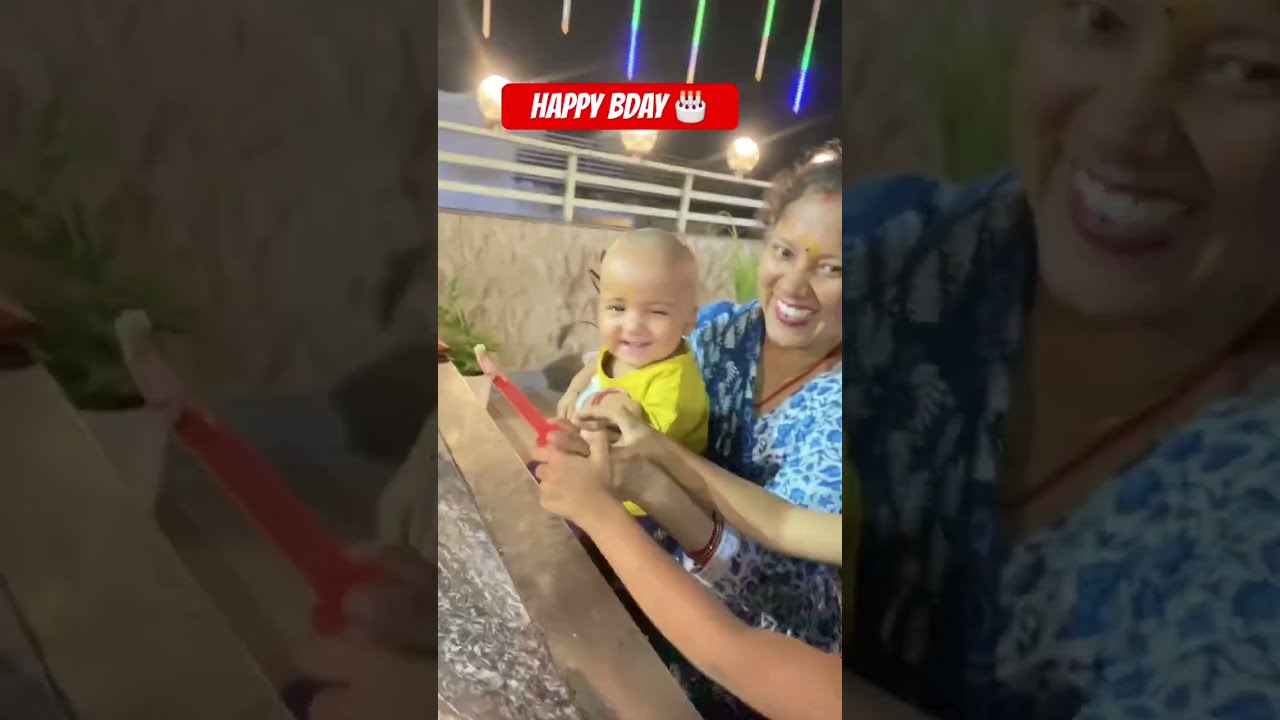In the image, a smiling woman with caramel-colored skin and curly dark brown hair cradles a cheerful, bald baby at the center of the frame. The baby, dressed in a neon yellow shirt, appears to be winking and smiling, adding to the overall joyful ambiance. The woman is wearing a blue and white shirt; one side displaying a blue background with white floral print and the other side white with blue floral print. She also has a small yellowish dot between her eyebrows, possibly a bindi. A pair of hands from another person, who is partially out of the frame, reaches in from the right side to hold the baby's hands. The setting includes a table in the bottom left and another person partially visible in the bottom right. Above them, a wall with a divider can be seen, and the top of the image features text reading "Happy B-Day" alongside lights, suggesting a festive atmosphere. The scene is colorful with visible shades of gray, black, brown, red, lime green, blue, purple, and green, hinting that the image might be a screenshot from a mobile app, possibly taken outdoors in a third-world country. The woman also sports a red necklace, adding to the vibrant setting.